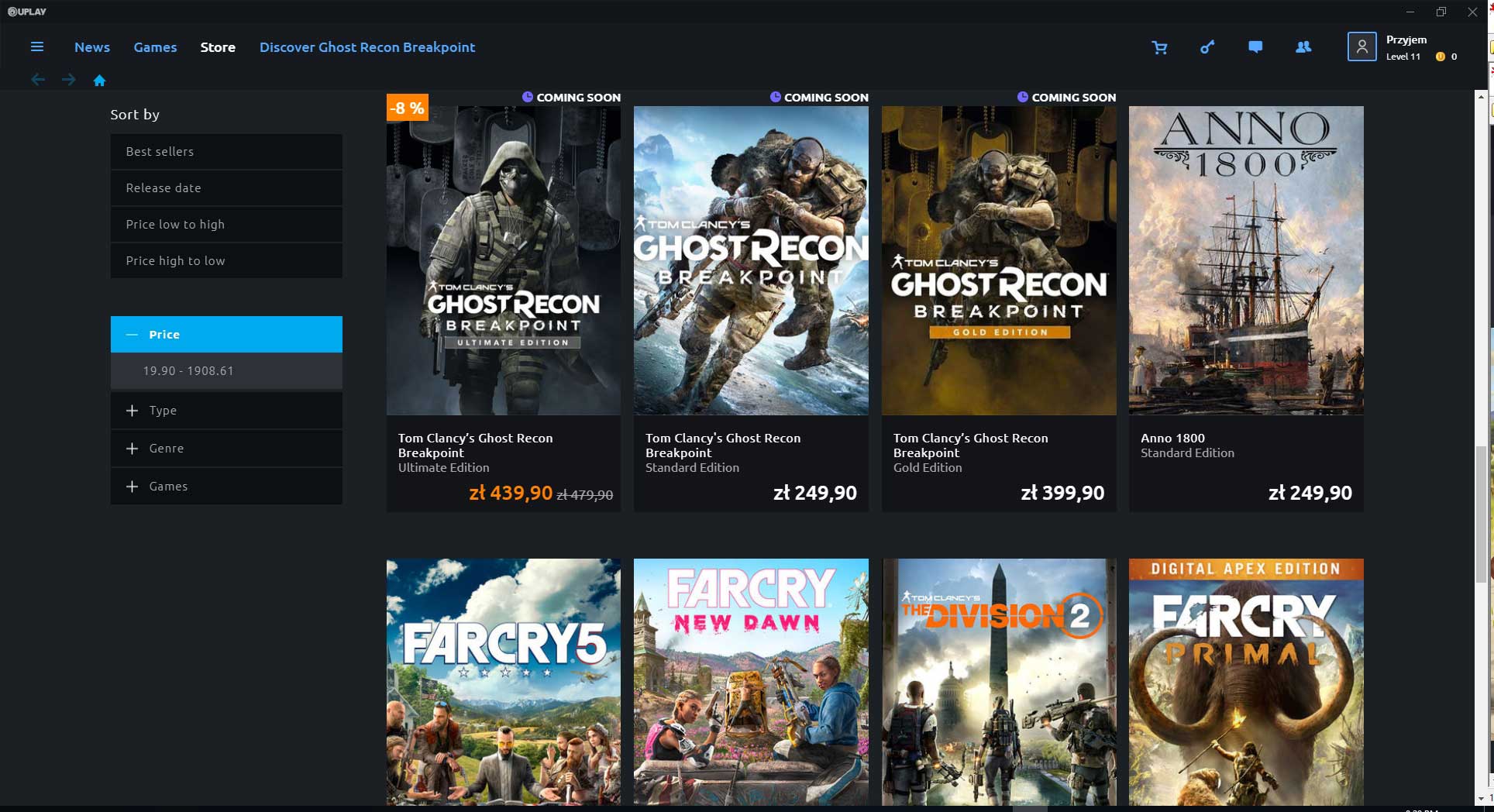Here we have a screenshot of a digital storefront displaying an array of video game titles. The interface is predominantly black, providing a sleek, modern look. Across the top of the screen are categories such as "News," "Games," "Store," "Discover," and "Ghost Recon Breakpoint," accompanied by a shopping cart icon, a chat icon, and a user profile icon. 

On the left-hand side, there is a column featuring a "Sort By" dropdown menu with various filtering options that are not fully legible in the screenshot. Below this, there are additional categories, again too small to decipher clearly.

In the main section, eight distinct video game covers are displayed in a grid arrangement. The detailed information for each game is as follows:

1. **Ghost Recon Breakpoint**: Priced at ZL43990, this cover features a dramatic illustration related to the game.
2. **Ghost Recon Breakpoint**: Another version priced at ZL24990, showcasing two soldiers, illustrating the subtitle "Tom Clancy's Ghost Recon Breakpoint."
3. **Ghost Recon Breakpoint**: Priced at ZL39990, this cover also displays two soldiers, possibly in an emotional embrace.
4. **Anno 1800**: Priced at ZL24990, this game cover showcases an old-fashioned sailing ship, capturing the historical essence of the game.

In the bottom row:
5. **Far Cry**: This cover shows a group of people standing in a valley under a blue, cloudy sky, emphasizing a sense of adventure.
6. **Far Cry New Dawn**: Priced similarly, it depicts individuals in a scenic, rocky foreground with a vibrant blue sky, suggesting a continuation or spin-off of the Far Cry series.
7. **The Division 2**: This features three soldiers with a backdrop that includes what appears to be a missile or rocket, hinting at an action-packed narrative.
8. **Far Cry Primal - Digital Apex Edition**: Highlighted with a dramatic picture of a large mastodon-like creature, indicating a prehistoric setting. 

Overall, the interface is designed to draw attention to the diverse range of games available for purchase, with each cover offering a glimpse into the unique worlds and stories they contain.